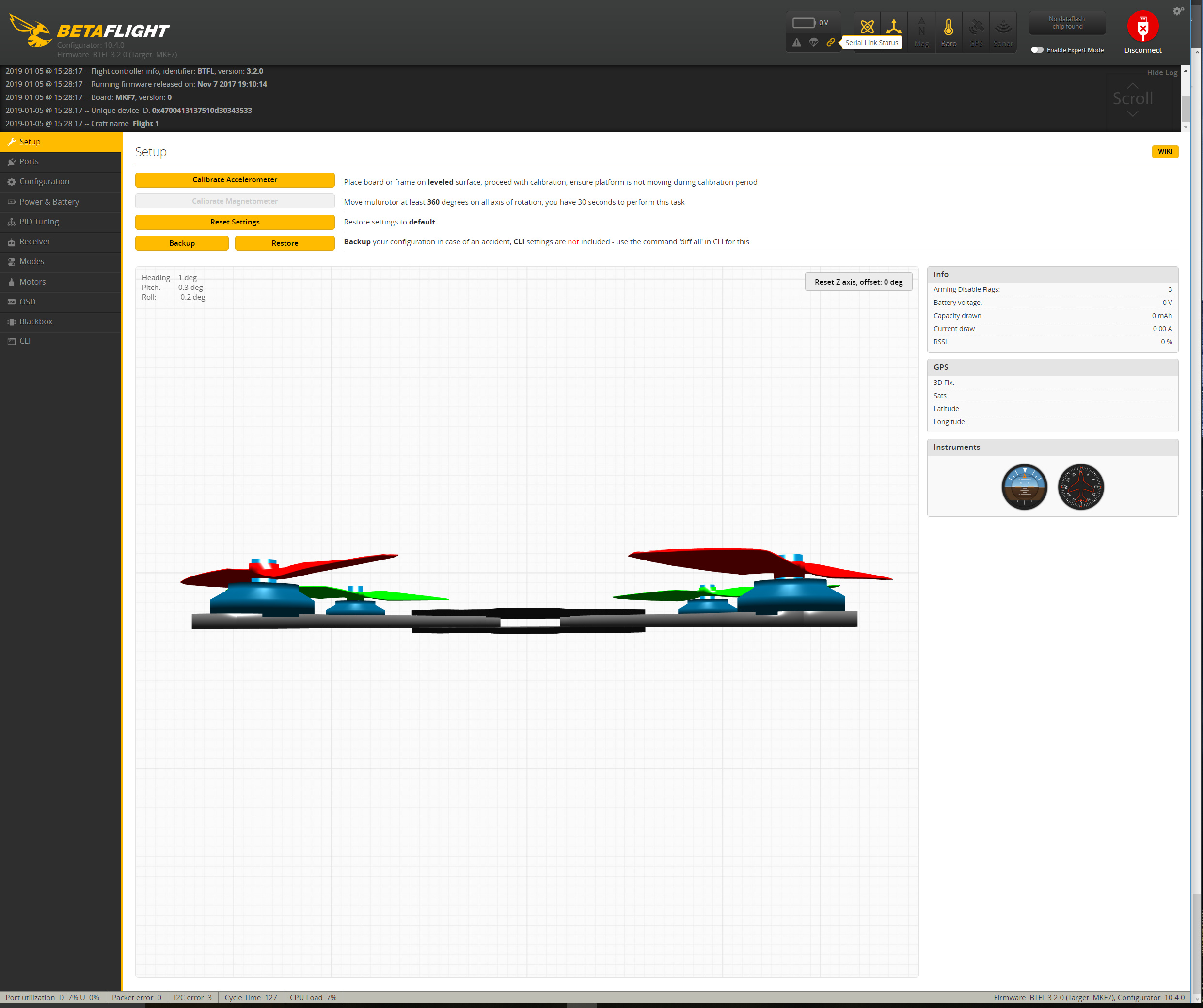The image displays a screenshot of a configuration interface for a drone, specifically within the BetaFlight software. At the top, the BetaFlight logo is prominently visible, featuring a cartoon bee that appears ready to sting, symbolizing agility and sharpness. The word 'Beta' is highlighted in yellow, while 'Flight' is in white, making it visually striking. 

In the 'Setup' section, which is highlighted in yellow, various calibration and configuration options are listed. The text 'Calibrate Accelerometer' is clearly visible, suggesting options for fine-tuning the drone's sensors. Further down, options such as 'Reset Settings' and 'Backup and Restore' are also highlighted in yellow, indicating essential functionalities available to the user.

The image also showcases a digitally rendered model of a flying device, likely a drone. This drone appears to have a teal-colored body with four propellers, two of which are green and two white. The visual presentation suggests that the interface is user-friendly and intuitively designed for drone enthusiasts and professionals.